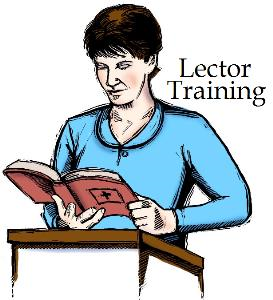In this hand-drawn illustration, a white woman with short brown hair, appearing to be around 30 to 35 years old, stands behind a wooden lectern. She is dressed in a blue, long-sleeved shirt featuring a high, rounded collar reminiscent of a Peter Pan style. The focus of the image is her holding an open, thick book with both hands; the book has a reddish, rose-colored cover displaying a cross symbol. Her eyes seem to be either closed or looking downward as she reads. The background of the image is completely white, and in the top right corner, the text "Lecter Training" is written in black letters. The image captures a serene and focused moment of the woman engaging with the book, likely the Bible.